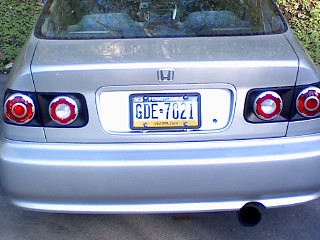The photograph captures the back end of a silver Hyundai sedan parked amidst greenery with visible grass and dirt. The focal point is the Hyundai logo in silver prominently displayed on the back. The vehicle features four uniquely designed taillights and brake lights. Each light is encased in a cool, gear-like silver design with red and white hues, set against dark black squares. The exhaust pipe is visible on the lower right side below the bumper. A Pennsylvania license plate, marked GDE 7021, is centrally located and bordered by a black license plate frame. The plate includes a sticker on the top left corner. Additionally, the image shows the car's back window and a bit of the interior, also silver, adding to the overall sleek appearance of the vehicle.